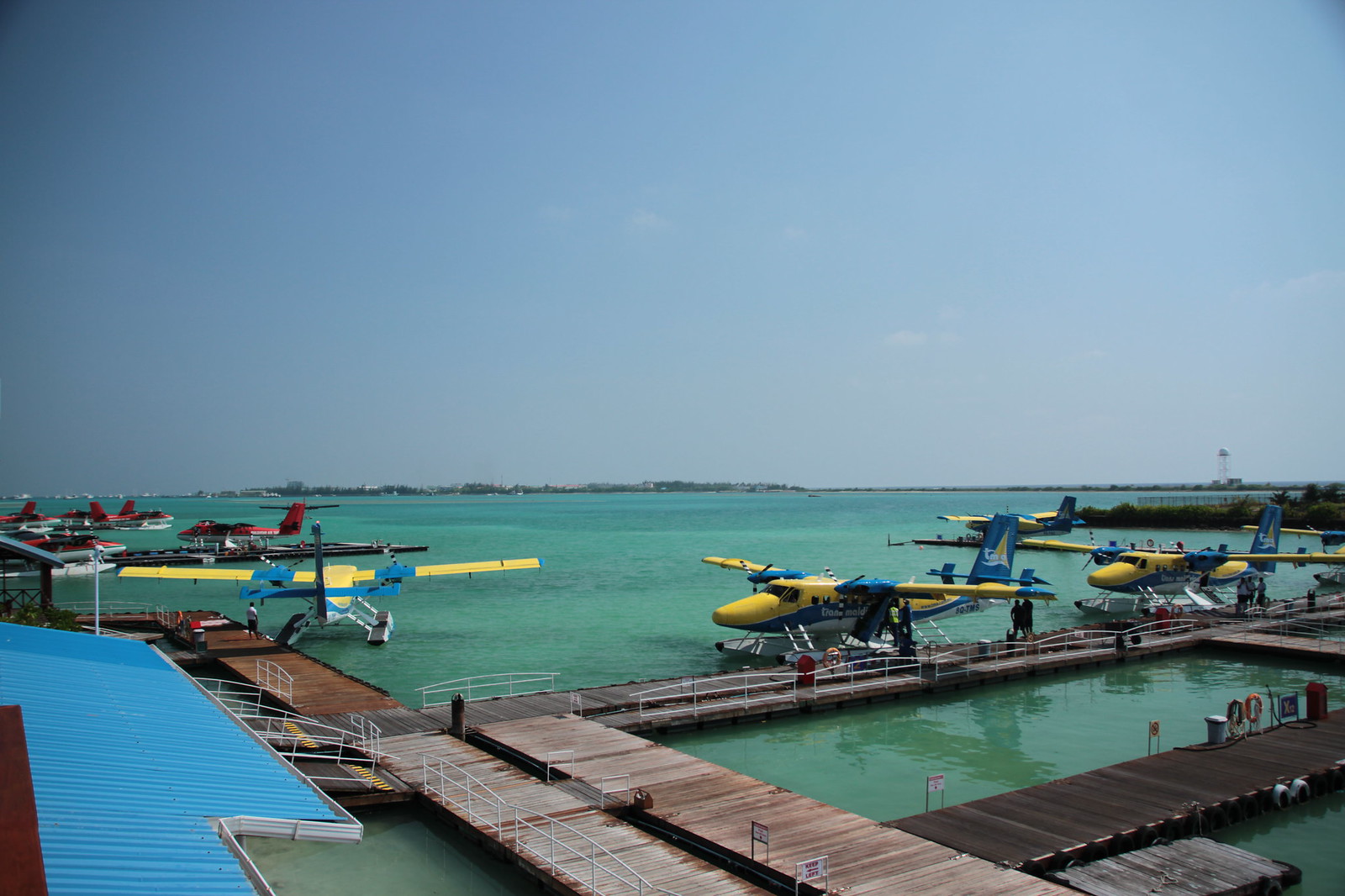The image captures a vibrant and busy hydroplane facility, characterized by several yellow and blue hydroplanes docked along a grid of intersecting boardwalks. These walkways, likely leading to a commercial establishment, connect to planes seemingly used for tourist flights, perhaps over the nearby islands. Four hydroplanes of the same yellow and blue design are prominently featured, while a separate section on the left shows additional red hydroplanes. The water beneath the planes is a striking green, suggesting a shallow depth or possible shadows. On the left, the edge of a blue-striped roof is visible, hinting at an adjoining building. Beyond the facility, the horizon reveals a glimpse of distant lands separated by water, under a light blue sky adorned with wispy clouds. To the right, a tall structure such as a lighthouse punctuates the distant landscape.